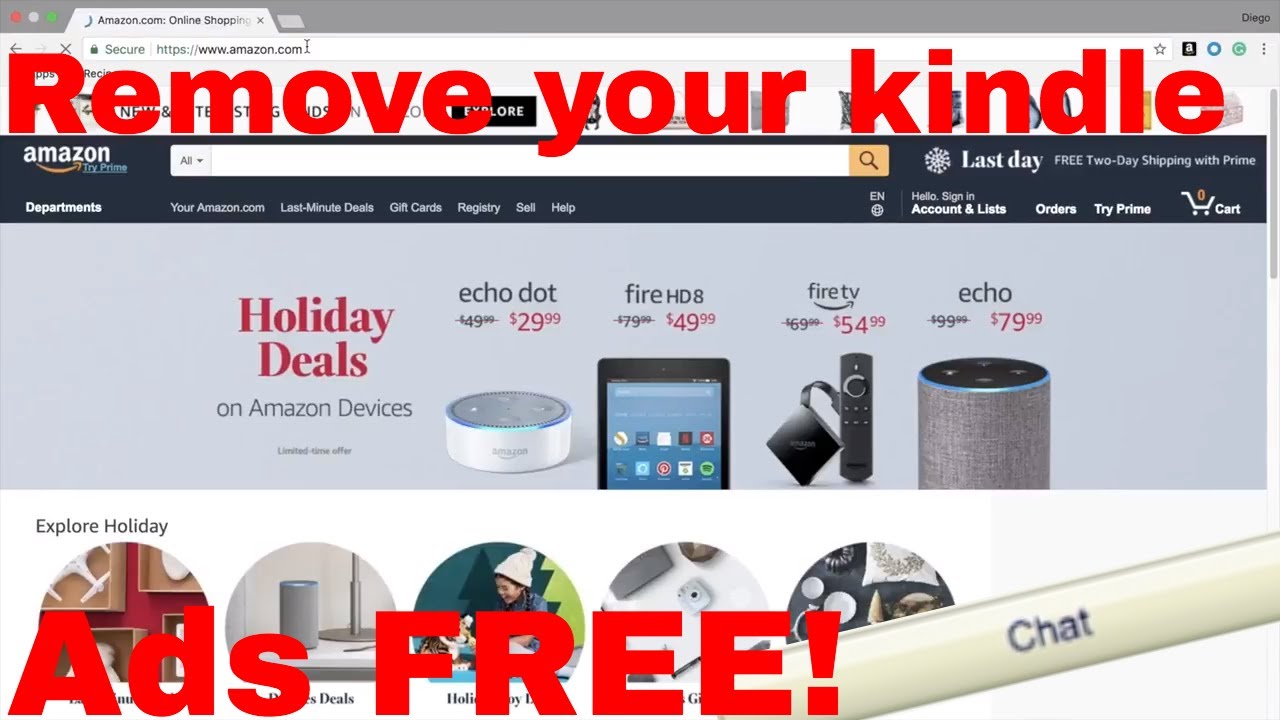The image displays a screenshot from the Amazon.com website. At the top, there is a gray browser bar indicating the URL "https://www.amazon.com" with browser elements including a left arrow, an 'X,' and a star icon. Below this, bold red text prominently states “Remove your Kindle.”

Beneath the browser bar, a black navigation bar displays the Amazon logo, the word "Prime," and several menu options such as "Departments," "Search," and the category "All." A promotional banner informs users about "Last day free two-day shipping with Prime," followed by navigation links for "Your Amazon.com," "Last Minute Deals," "Gift Cards," "Registry," "Sell," "Help," "Account & Lists," "Orders," "Try Prime," and "Your Cart."

A large blue banner featuring the heading "Holiday Deals" in red highlights special offers on Amazon devices. The deals include:
- Echo Dot for $29.99
- Fire HD 8 for $49.99
- Fire TV for $54.99
- Echo for $79.99

The prices are emphasized in red text. Directly below, a white box urges users to "Explore Holiday," with the text "Ads free" highlighted in red. The box also includes a long button labeled "Chat."